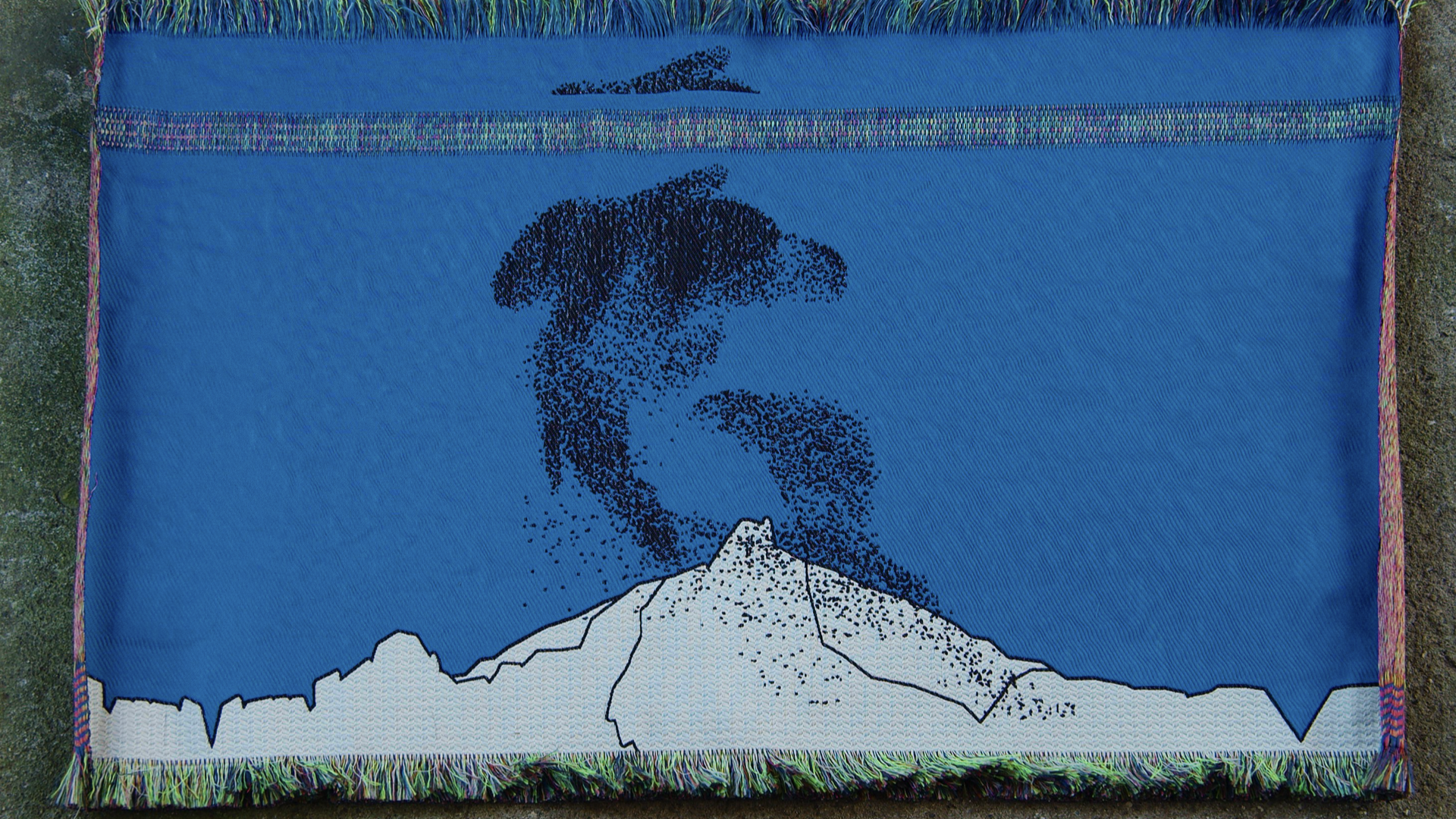The image depicts a blue rug lying on a green carpet that resembles the color of a putting green. The rug features detailed and intricate elements, including fringes on both the top and bottom edges. The primary design on the rug includes a section at the bottom with a lighter blue or grayish mountain-like shape that peaks in the center and tapers off towards the edges. Additionally, there are black elements on this section, possibly representing either trees or sea creatures. The main body of the rug showcases a series of dots forming the shape of a dolphin, with a more detailed outline, and another less detailed dolphin below it. There is also a stripe or design element running horizontally across the top of the rug, which could be interpreted as stitching. The rug appears somewhat thin and has a soft, textured appearance, potentially hinting at its use as a decorative piece or a soft mat.